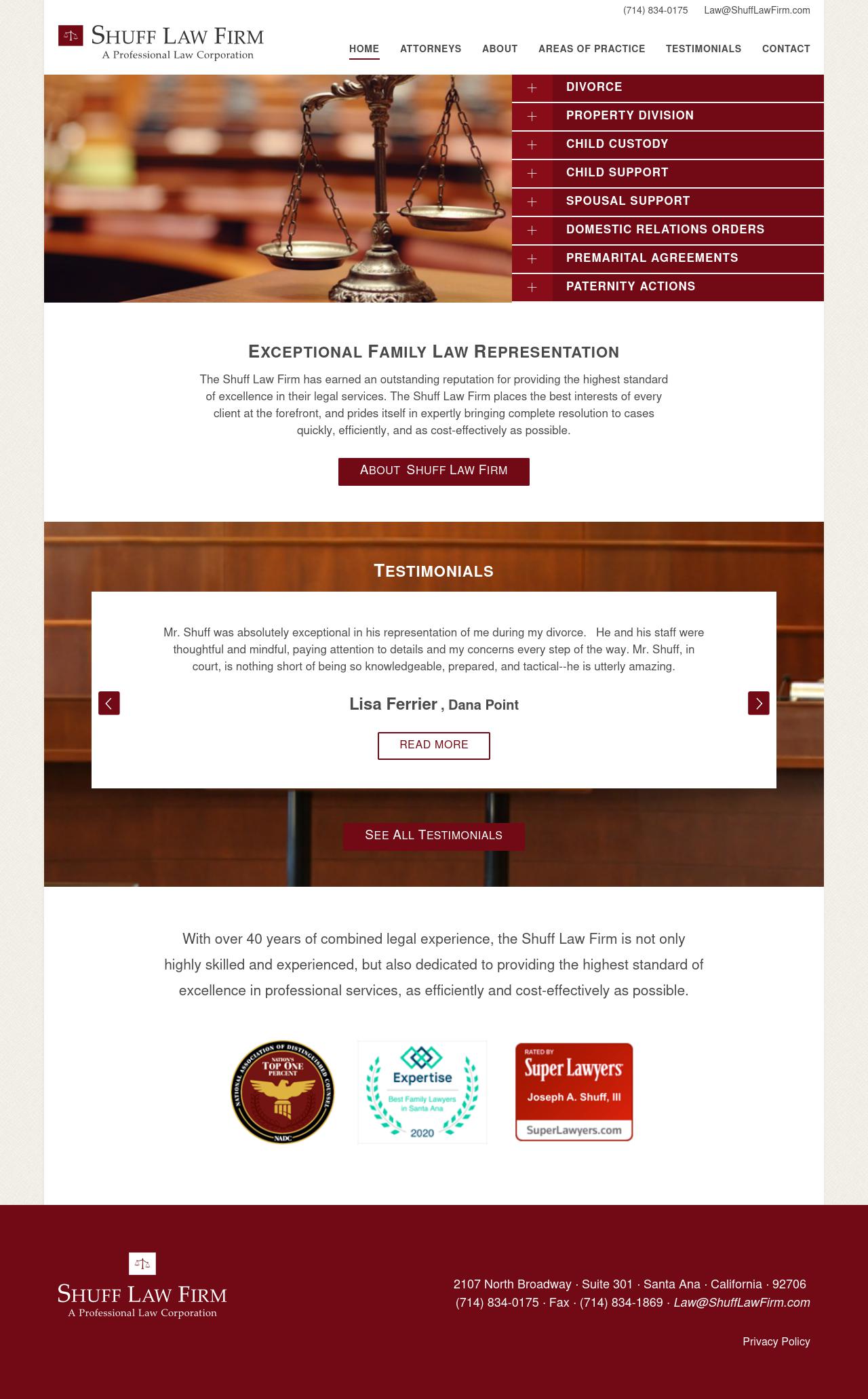The image depicts a website screenshot set against a beige-white background. In the upper left corner, there is a professional logo for "Shuff Law Firm, a Professional Law Corporation." The logo consists of a red box featuring a scale icon, symbolizing justice. Adjacent to the logo, the navigation menu items are arranged horizontally: Home, Attorneys, About, Areas of Practice, Testimonials, and Contact.

Dominating the left side of the screenshot is a color photograph of a brass, vintage-style scale, emphasizing the firm’s commitment to justice and balance. To the right of the photograph, white text on a dark red background lists the firm’s areas of expertise: Divorce, Property Division, Child Custody, Child Support, Spousal Support, Domestic Relations Orders, Premarital Agreements, and Paternity Actions.

At the bottom of the screenshot, a testimonial section is prominently featured within a white box. The testimonial reads: "Mr. Shuff was absolutely exceptional in his representation of me during my divorce. - Lisa Ferrer, Dana Point." This endorsement highlights client satisfaction and the firm’s expertise in handling divorce cases.